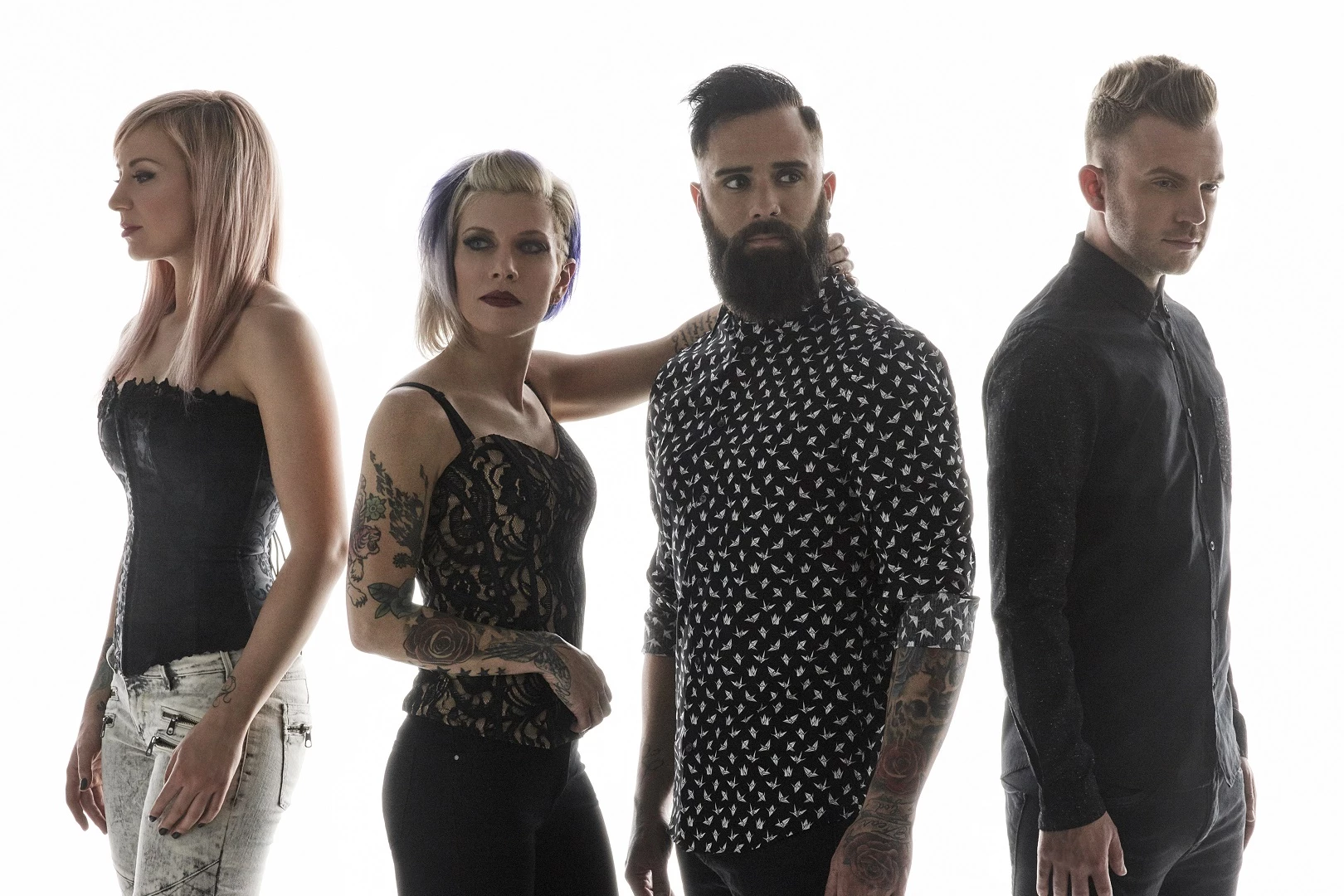This high-fashion modeling photograph features four individuals, evenly spaced and centered against a pristine white background. The composition includes two women and two men, all of whom appear to be Caucasian and are adorned in modern, stylish attire. 

On the far left stands a blonde woman with straight, dirty blonde hair cascading just above her breasts. She wears a dark halter top akin to a bustier and white, acid-washed jeans, her arms hanging naturally by her sides with dark fingernail polish adding a sleek touch.

Next is a second woman with short, platinum blonde hair that brushes her neck and lips painted a bold red. She's adorned in a lacy, see-through sleeveless top paired with black jeans. Her right arm, bent at the elbow, prominently displays intricate black tattoos that extend from her shoulder to her wrist. She stands in profile, facing right but tilting her head slightly left.

To her right, a bearded man is captured with a commanding presence. His dark hair and substantial beard frame a face that gazes slightly left. He dons a black button-down shirt patterned with white bird-like shapes and paired with black pants. His shirt is untucked, and his sleeves rolled up, revealing a left arm completely sleeved with tattoos.

On the far right, another man with short brown hair stands in profile, facing right. He wears a dark jacket over a black button-up shirt, paired with very dark gray or black jeans. His casual stance has his right arm hanging comfortably at his side as he glances slightly downward.

Set against the minimalist white backdrop, these individuals are likely showcasing contemporary fashion, their distinct styles and confident postures suggesting a high-fashion advertisement.